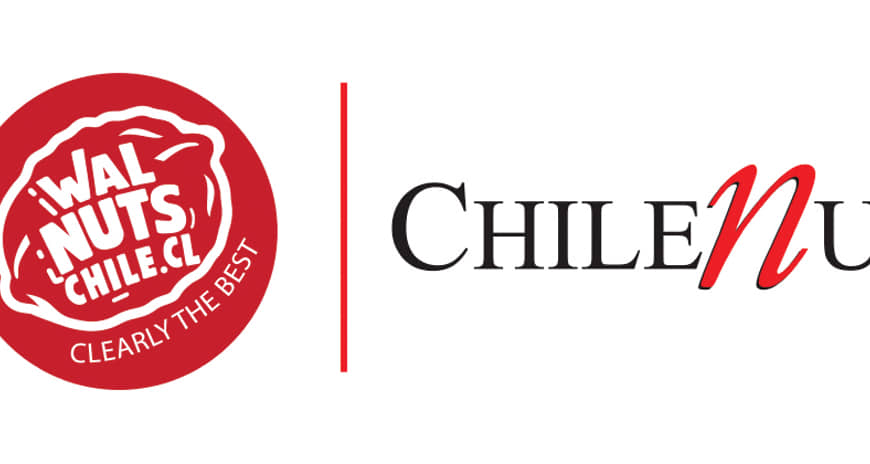The image depicts a business logo set against a white background. On the left side, there is a large red circle containing a white walnut shape with the text "walnutschile.cl" in white letters inside the walnut. The walnut has a white outline with detailed white lines within that give it a 3D effect. Below this walnut, the phrase "Clearly the Best" is inscribed in white font. To the right of the red circle, a thick red vertical line serves as a separator. Beyond this line, the text "Chile" is written in black capital letters followed by a large, cursive red letter "N" and a black letter "U." The rest of the text is presumably cut off. The overall design suggests the logo represents a promotional or branding image related to walnuts from Chile.